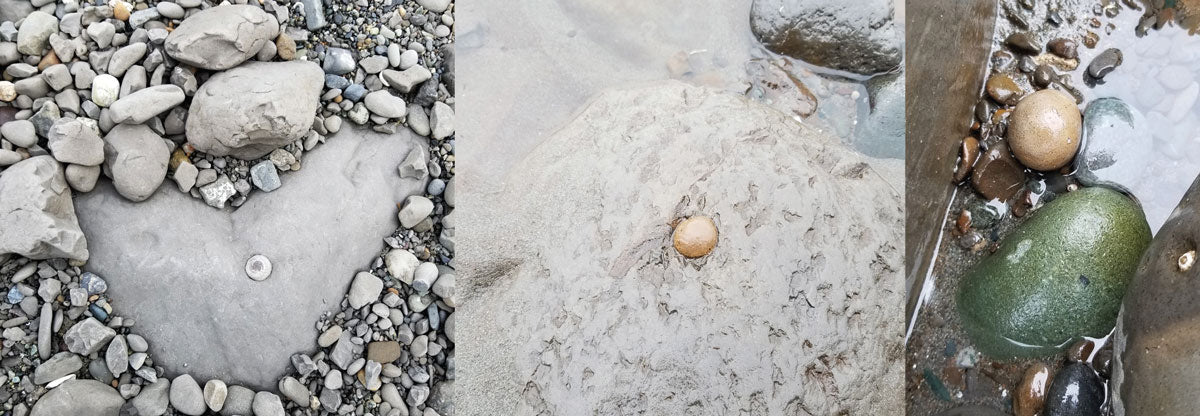The image is a horizontally aligned, rectangular photograph divided into three sections: two squares on the left and center, and a vertical rectangle on the right. The left section features a variety of smooth, dry stones and pebbles, predominantly in gray tones. The focal point is a large, flat, heart-shaped stone that is light gray in the middle, surrounded by larger stones on the top and left and a mix of smaller gravel-like stones.

In the middle, there's a textured beige surface resembling petrified mud with a small, gold-colored rock in its center. The top right corner of this section appears wet and features what looks like a frog.

The right section displays a green, possibly moss-covered stone that mimics the top of a frog, with the same gold ball seen in the middle section just above it. The surrounding area contains various other pebbles and appears wet, suggesting the presence of a stream or water source nearby. The overall composition captures a range of stone types, from smooth and pale to rough and textured, unified by the moist and dry elements across the sections.